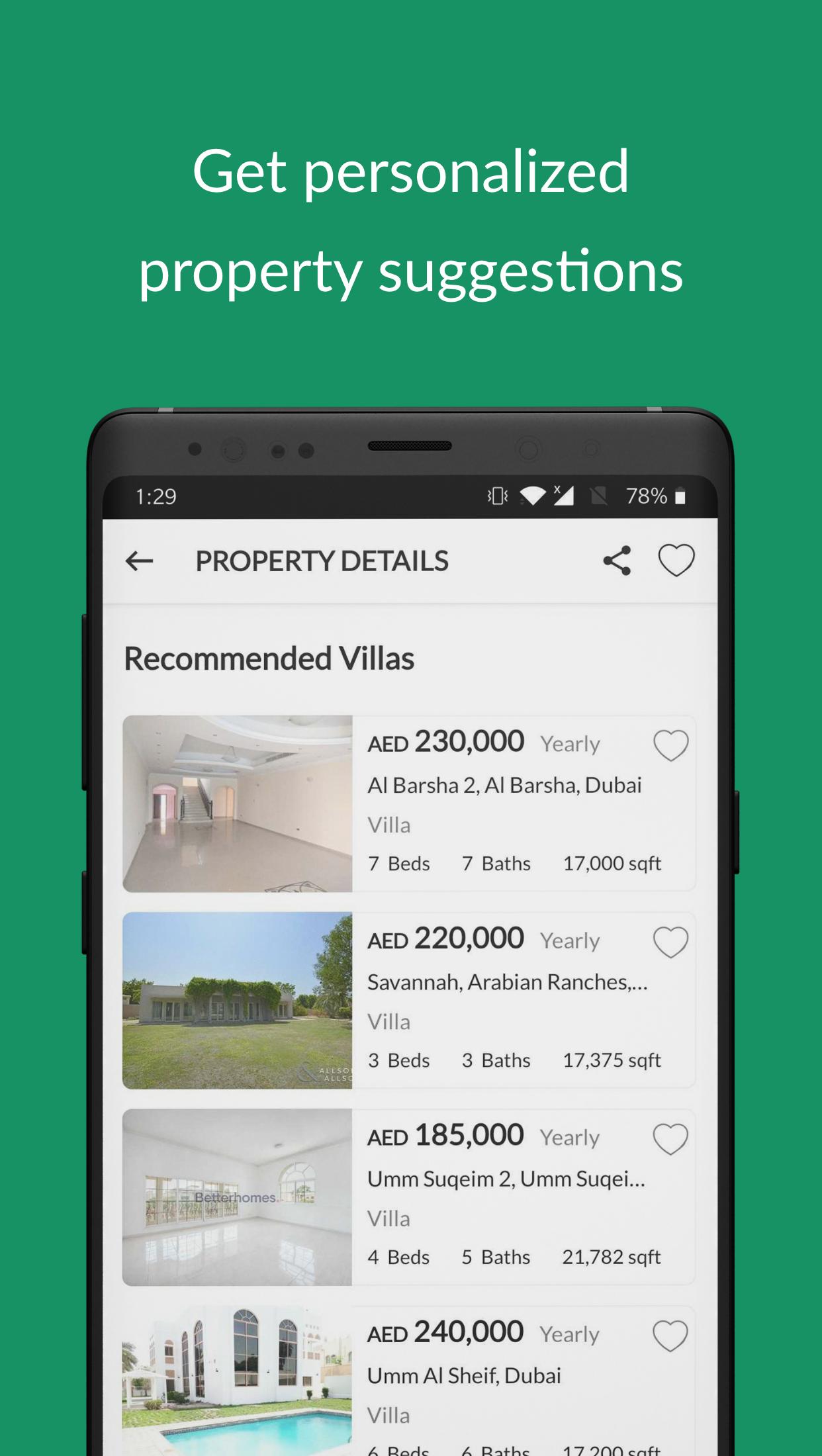A vertical, rectangular image with a vibrant green background that frames the central content. Dominating the middle section, starting from about two-thirds of the way up and extending downward, is the depiction of a smartphone screen. Positioned above the smartphone, in crisp white text, is the message: "Get personalized property suggestions."

The smartphone display showcases detailed property listings under the title "Property Details" followed by the heading "Recommended Villas." Four distinct villa options are presented, each accompanied by a thumbnail image on the left and descriptions on the right. 

1. The first listing, titled "Al-Barsha II, Al-Barsha Dubai Villa," features seven bedrooms, seven bathrooms, and covers an area of 17,000 square feet.
   
2. The second option, listed at AED 220,000 yearly, is identified as the "Savannah Arabian Ranches Villa," offering three bedrooms, three bathrooms, and spanning 17,375 square feet.
   
3. A third property, priced at AED 185,000 yearly, is the "Bound Sukhum II Villa," which includes four bedrooms, five bathrooms, and an expansive 21,782 square feet of living space.

This well-organized layout suggests someone is exploring various rental villas, emphasizing convenient and personalized property suggestions through the displayed smartphone interface.